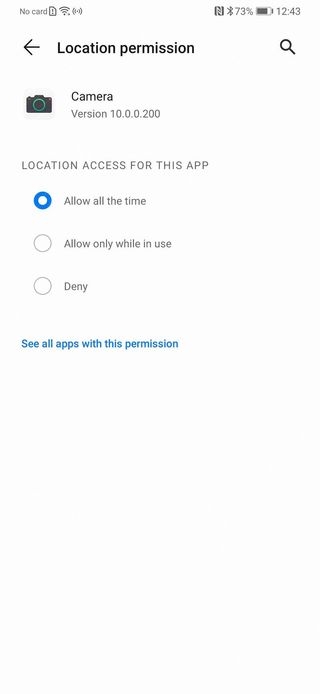The image shows the camera app's settings screen on a smartphone. At the very top, in tiny gray text on the left, it states "No card," indicating the absence of a memory card. To the right of this, there are icons indicating mobile signal strength and battery usage at 73%, with the current time displayed as 12:43.

Directly below this, larger black text reads "Location permission." To the left of this text is a left-pointing arrow, and to the right, a search button. 

Beneath this heading, there is a camera icon next to the word "Camera" in black text, with "version 10.0.0.200" listed underneath in gray text. Further down, it mentions "Location access for this app" in gray text. 

There are three permission options: 
1. "Allow all the time" (which is selected, indicated by a blue and white highlight),
2. "Allow only while in use,"
3. "Deny."

At the very bottom, in small blue text, it says "See all apps with this permission."